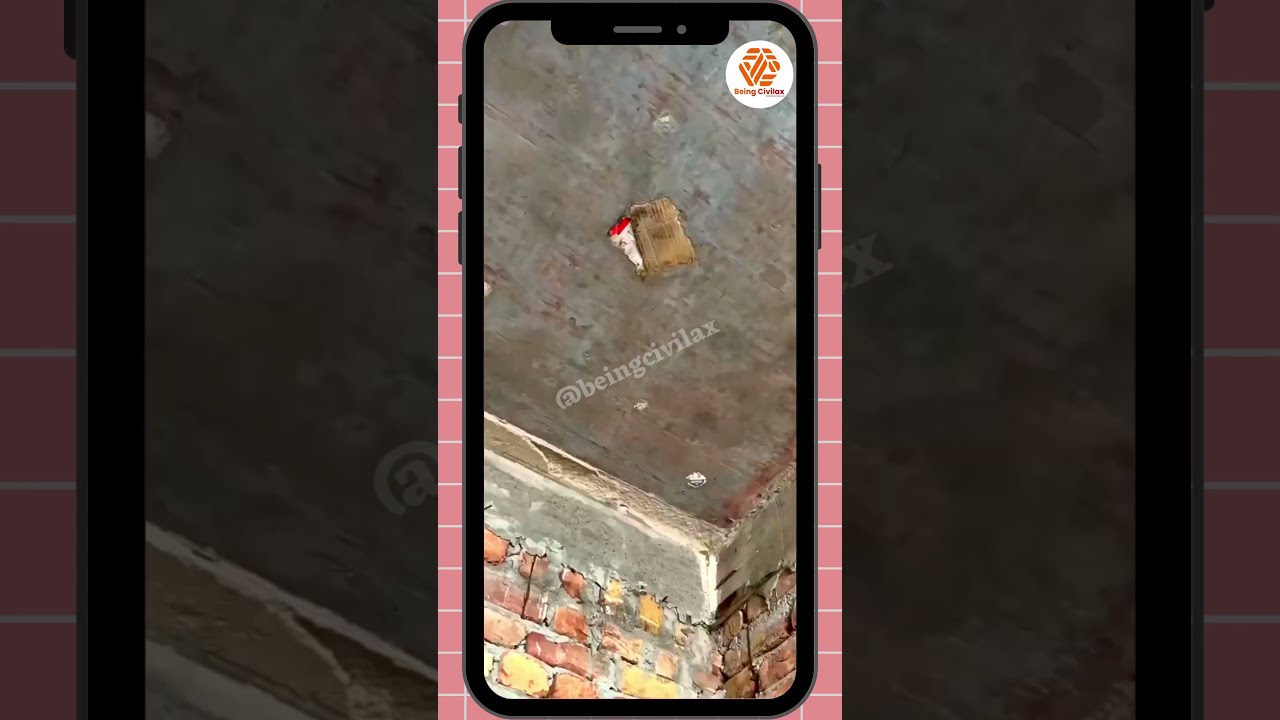In this photograph, the central focus is a vertically positioned black cell phone displaying an image of a brick wall corner and ceiling. This phone is placed within a vertical strip set against a larger horizontal rectangle. The background of the vertical strip is composed of pinkish, salmon-colored bricks. On the phone display, the image shows a brick wall meeting a smooth concrete ceiling, with a brown and white object placed in the middle of the ceiling, resembling some sort of decorative item or possibly food. In the top right corner of the phone's screen, there is a circular orange logo with a white border, containing the text "CIVIL X". Additionally, a gray watermark reading "@beingCIVILX" is positioned in the middle of the image on the phone. The entire horizontal background of the main image features a slightly blurred, close-up depiction of the pinkish brick pattern from the vertical strip, creating a layered and cohesive design. The overall setting suggests an advertisement or promotional material for "beingCIVILX."